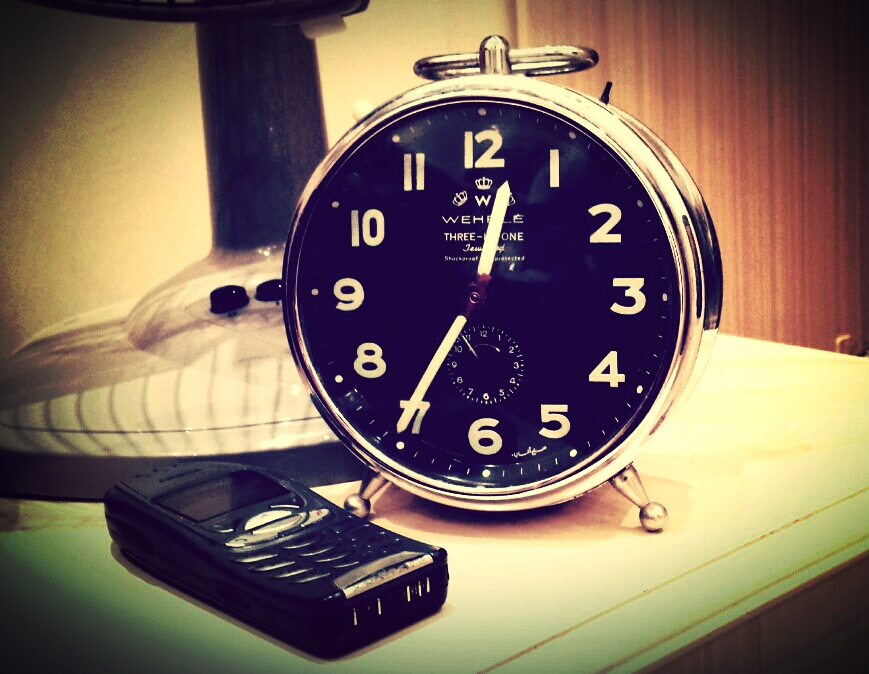This photograph features a side table in a room, artistically filtered to evoke a vintage aesthetic. On the pristine white tabletop, a white lamp with black buttons stands in the background, casting a subtle glow that adds to the retro ambiance. In the foreground, a classic black Nokia cell phone with silver buttons is prominently displayed, evoking a sense of nostalgia. To the right of the cell phone, in front of the lamp, sits an elegant vintage alarm clock. This circular clock, perched on two silver feet, has a silver rim that perfectly complements its design. The clock's face is black, with white numbers and notches offering a striking contrast. The white clock hands point to the time, which reads 12:35, further enriching the timeless vibe of the entire scene.